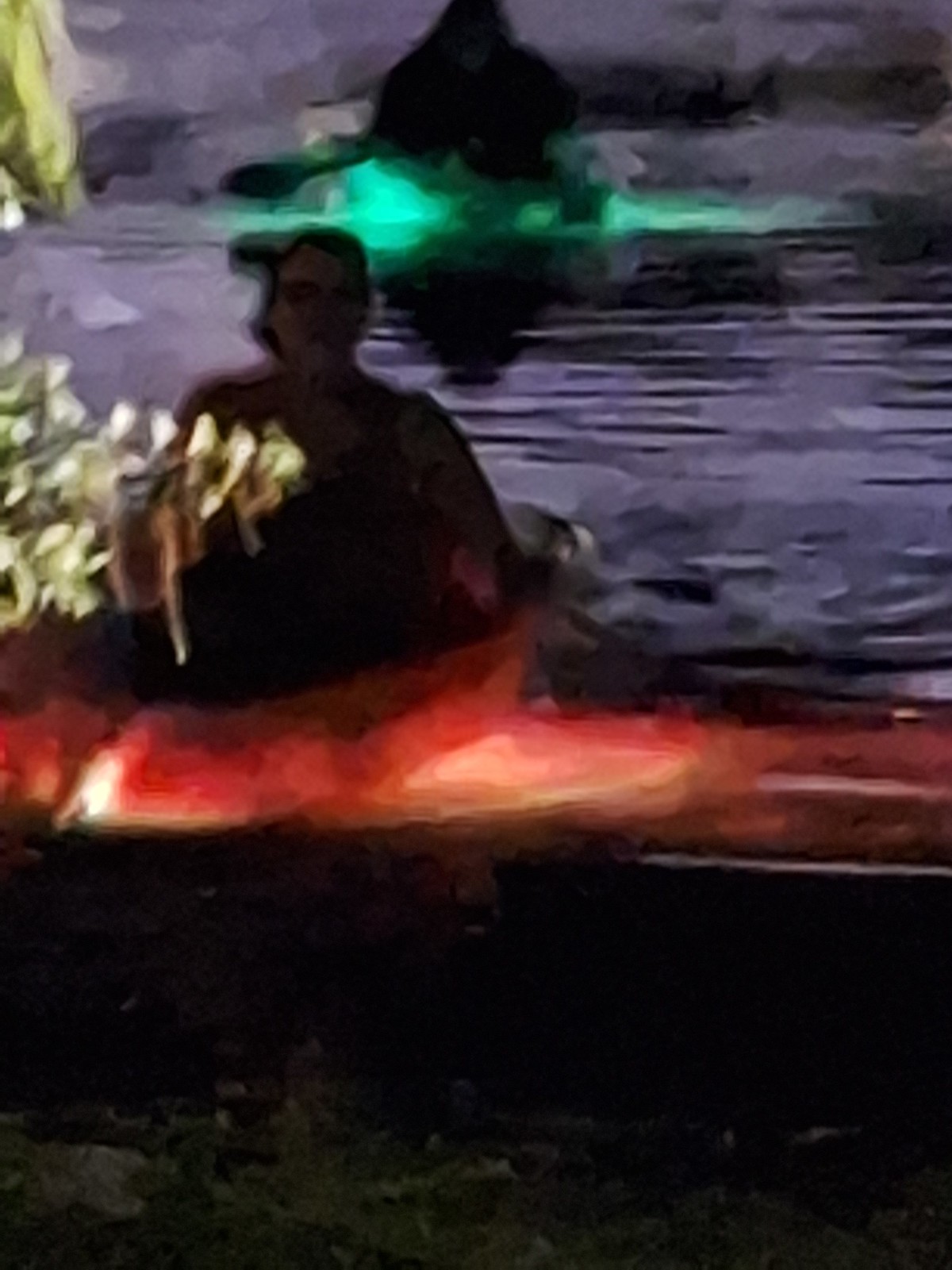This nighttime outdoor scene, possibly an oil painting or digitally altered photograph, features two individuals in separate, illuminated kayaks on dark water. The first kayak, brightly lit in green, contains a shadowy figure whose specific features are indiscernible. The second kayak, illuminated in red and pink hues, houses a person in a baseball cap and t-shirt, possibly a woman with short hair and glasses, facing forward. The water, appearing dark with purplish-gray tones, contrasts with the vibrant lights of the boats. Tree branches with leaves extend into the frame from the left, adding to the scene's depth and detailing.